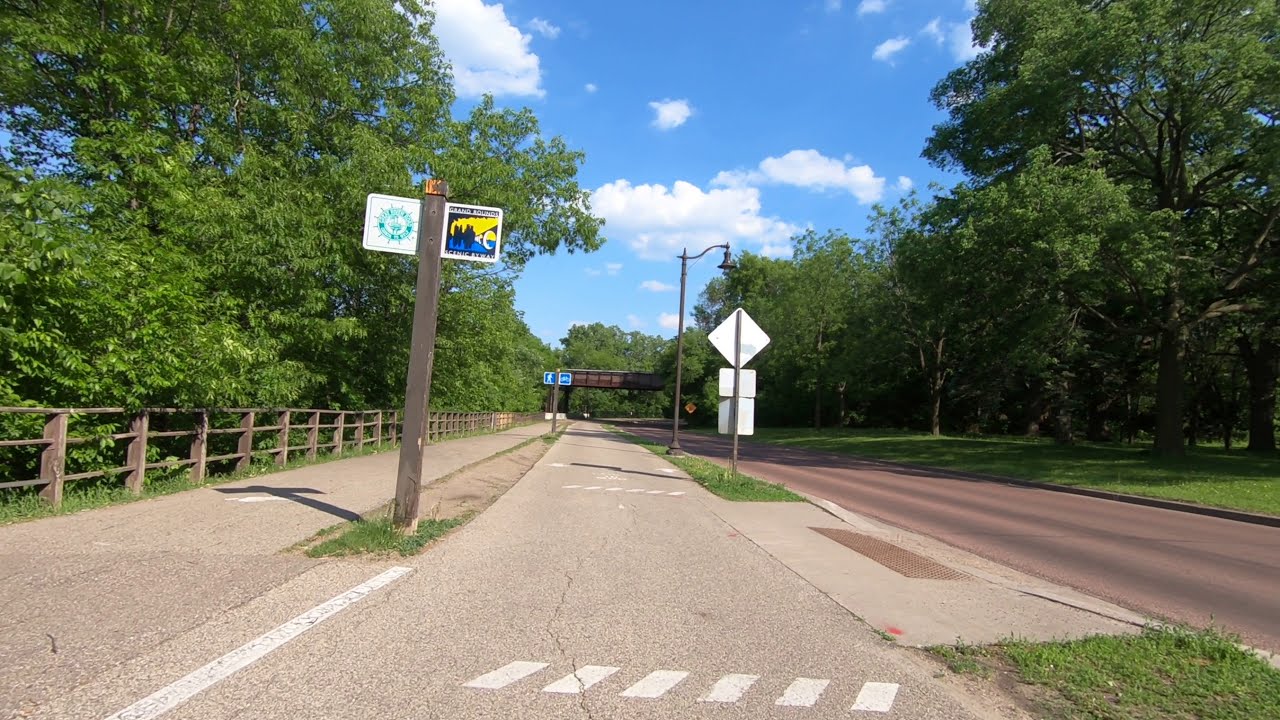This outdoor daytime scene captures a vacated road flanked by verdant trees and lush greenery. The image is dominated by two parallel roads—the right one being a darker gray and the left a lighter gray, marked with white stripes. A prominent crosswalk runs through the foreground. On the left side, a low, wooden three-tiered fence stretches next to dense, fluffy green foliage that extends to the horizon. On the right side, a well-maintained lawn spotted with large, leafy trees contributes to the vibrant greenery. Centered in the image is a significant street sign post adorned with a diamond sign and two rectangular signs beneath it, supported by a tan, old-fashioned light post. In the distance, a bridge spans across the roads, surrounded by more lush trees, completing this pastoral roadside vista. The sky above is a brilliant blue, scattered with picturesque white clouds, emphasizing the serene beauty of the scene.